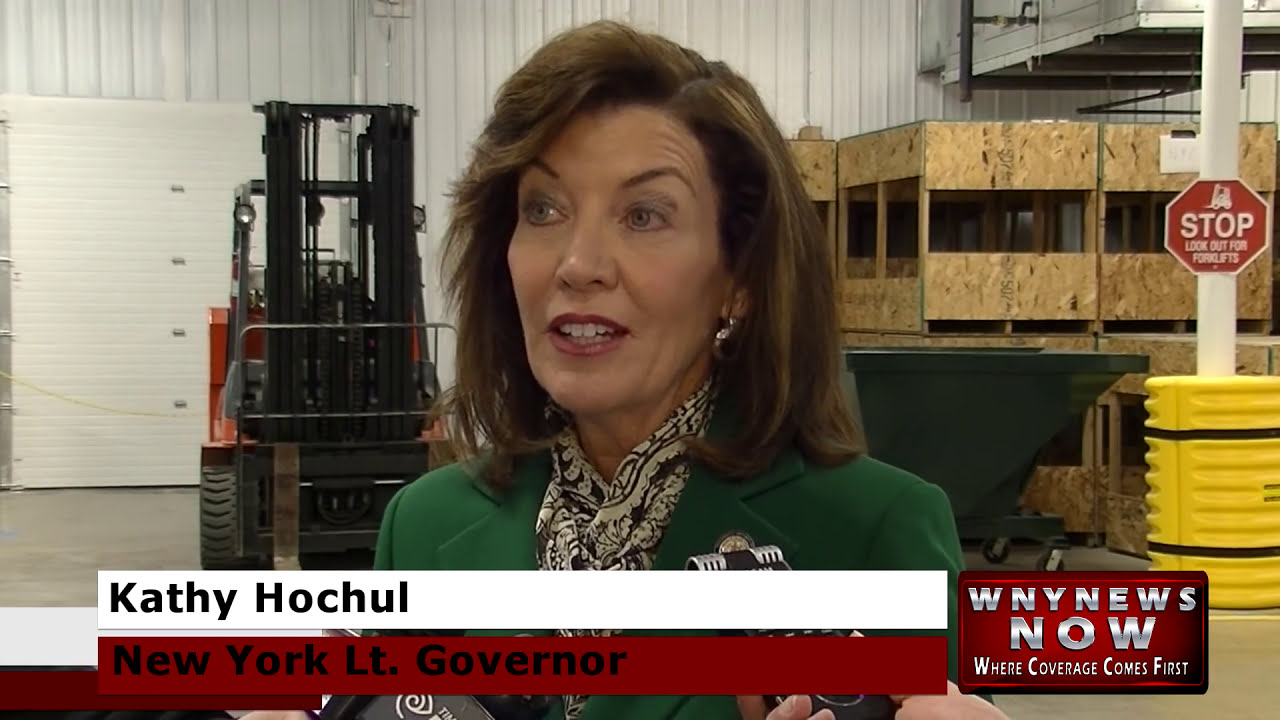This image features Kathy Hochul, the current Governor of New York, though she is pictured here during her tenure as the state's Lieutenant Governor. She stands centrally, occupying the bottom center portion of the photograph, and appears to be talking to an interviewer from a news channel. Hochul, a middle-aged white woman with shoulder-length dark brown hair parted slightly to the left, has highly arched eyebrows and wears deep burgundy lipstick. Her hair is styled down to her shoulders with an earring visible on her right ear. She is dressed in a green jacket over a high-necked, black and white printed blouse, and has a black and white paisley scarf draped around her neck.

In the bottom left corner of the image, a rectangular news banner in black letters reads "Kathy Hochul." Below this, in a similar long, red rectangular bar, it states "New York Lieutenant Governor." On the bottom right, another red rectangle banner displays "WNY News Now" in white letters, followed by the tagline "Where coverage comes first."

The background indicates a warehouse setting with elements of industrial equipment and storage. Behind Hochul's right shoulder is a forklift and a white-paneled wall. To her left, there are stacked pallets, wooden boxes, and a yellow area with a pole that includes a red "STOP" sign intended to safeguard the post from impact. The image also captures a yellow trash can and microphones' tips in front of Hochul.